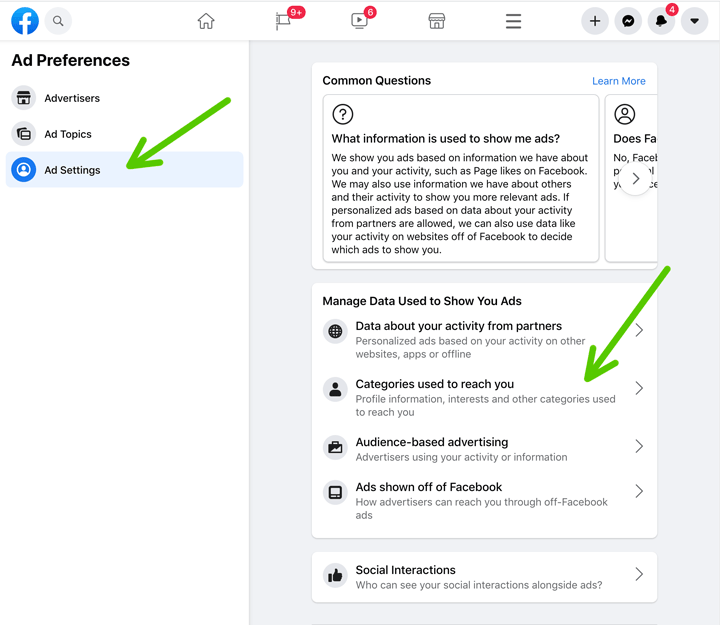This screen capture from Facebook displays a user navigating their ad preferences settings. In the top left corner, a blue circle with a white "F" prominently represents the Facebook logo. Across the top navigation bar, icons include a magnifying glass for search, a home button, and a flag with a red notification bubble indicating 9+ alerts. A video icon also displays a red notification bubble with the number 6, while on the far right, three stacked horizontal lines signify the menu options.

Down the left side of the image, "Ad Preferences" is labeled prominently in black bold lettering on a white background. Under this section, options listed include "Advertisers," "Ad Topics," and "Ad Settings." The user has selected "Ad Settings," highlighted by a bright blue circle. This selection is further emphasized by a green arrow pointing diagonally from the top right to the bottom left, directing attention to the ad settings.

On the right side of the page, a section labeled "Common Questions" features information on various ad-related topics. The questions include "What information is used to show me ads?", "Manage data used to show you ads," "Data about your activity from partners," "Categories used to reach you," "Audience-based advertising," "Ads shown off Facebook," and "Social interactions." Another green arrow, also pointing diagonally from the top right to the bottom left, highlights the "Categories used to reach you" option. In the upper right corner of this section, a blue "Learn More" link is available for users seeking additional information.